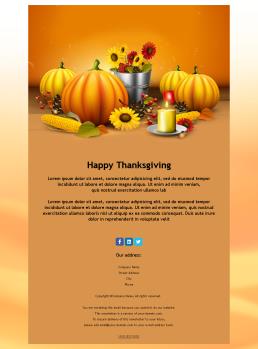A festive Thanksgiving display features an assortment of pumpkins, ears of corn, candles, and flowers illuminated by warm candlelight. The bottom of the image includes social media icons for Facebook, LinkedIn, and Twitter, along with an address, though the text is unfortunately illegible due to poor image quality. Visible colors in the scene include shades of yellow, gold, red, blue, and black text, evoking a rich autumnal palette. Despite the emergency watermark, the atmosphere remains celebratory and inviting.